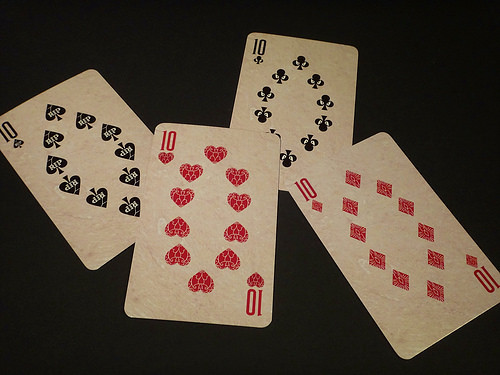This landscape-oriented photograph showcases a striking arrangement of four overlapping playing cards against a solid black background. Each card is partially obscured, creating a layered effect that draws the eye across the image. 

Starting from the left, the first card is the Ten of Spades. Positioned almost diagonally, its tip nearly touches the left-center edge of the frame, while the top is cut off by the photo's boundary. The Ten of Spades features ten spades arranged in a diamond pattern at its center.

Next, the Ten of Hearts is slightly overlaid on the Ten of Spades. This card extends to the bottom-center of the photo and covers part of the Spades card's back end. It displays ten heart symbols arranged similarly to the spades.

Overlapping the Ten of Hearts is the Ten of Clubs, which starts near the top-center and extends downward toward the bottom right. The clubs are arranged in the same central pattern as the previous cards.

The final card, the Ten of Diamonds, begins at the bottom right and extends toward the center, partially obscuring the lower part of the Ten of Spades. This card features ten diamonds arranged in a circular pattern.

Each card retains its unique watermark and suit while contributing to a cohesive and visually appealing composition.